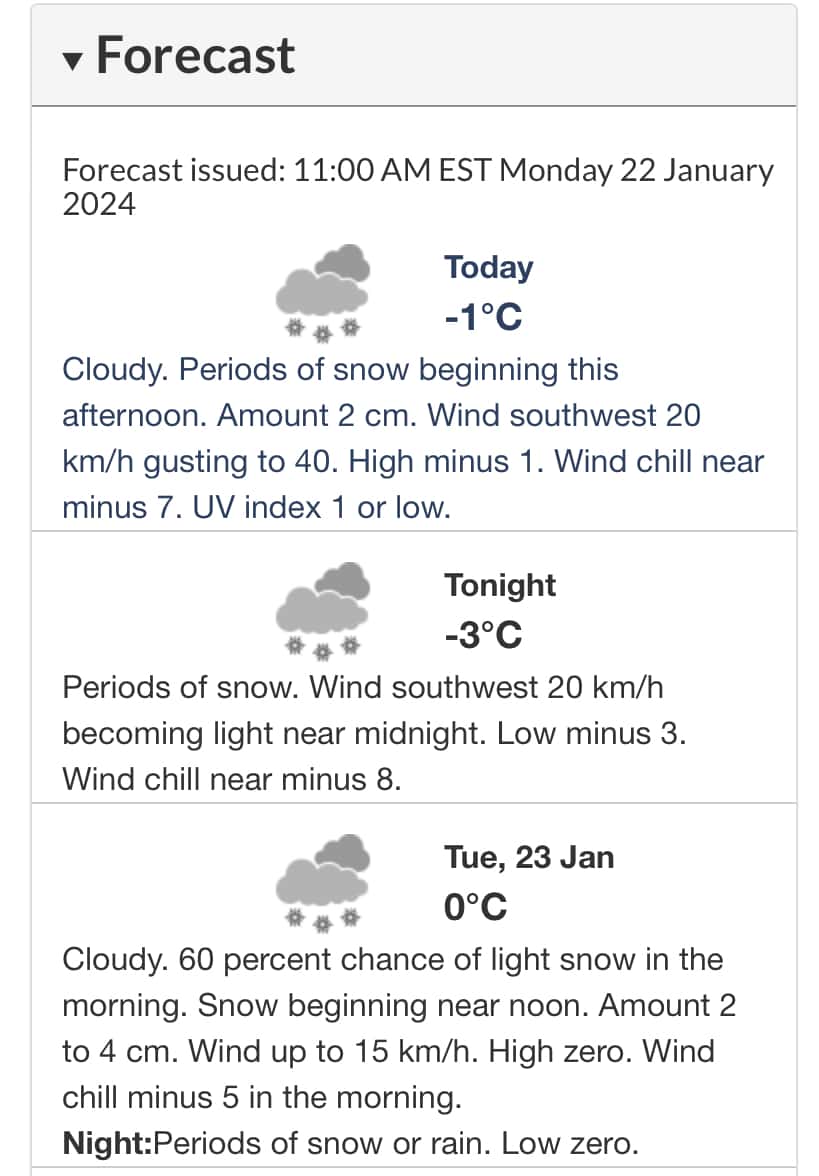This image displays a detailed weather forecast on a simple white background, providing information for the upcoming days.

At the top of the image, a gray bar contains the bold word "Forecast" with a drop-down box. Below this title, another line of text in smaller font reads, "Forecast issued 11 AM Eastern Monday, January 22, 2024."

The forecast is divided into three neatly separated sections by horizontal lines, creating a uniform appearance. Each section is displayed against a white background:

1. **Today (January 22)**
   - **Temperature:** -1°C, highlighted in blue
   - **Forecast:** Snowflakes icon indicating snowy conditions
   - **Description:** "Cloudy with periods of snow beginning this afternoon, accumulating about 2 centimeters."
   - **Wind:** Southwest at 20 kilometers per hour, gusting up to 40 kilometers per hour
   - **High:** -1°C
   - **Wind Chill:** Feels like -7°C
   - **UV Index:** 1 (Low)

2. **Tonight**
   - **Temperature:** -3°C
   - **Forecast:** Snowflakes icon indicating continued snow
   - **Description:** "Periods of snow with winds from the southwest at 20 kilometers per hour, calming late near midnight."
   - **Low:** -3°C
   - **Wind Chill:** Feels like -8°C

3. **Tuesday (January 23)**
   - **Morning Temperature:** 0°C
   - **Forecast:** Cloudy with a 60% chance of light snow in the morning and snow beginning near noon, accumulating 2 to 4 centimeters
   - **Wind:** Up to 15 kilometers per hour
   - **High:** 0°C
   - **Wind Chill:** Feels like -5°C
   - **Evening Forecast:** "Periods of snow or rain, with a low of 0°C."

The overall design is clear and easy to read, ensuring that all critical forecast information is readily accessible and visually organized.